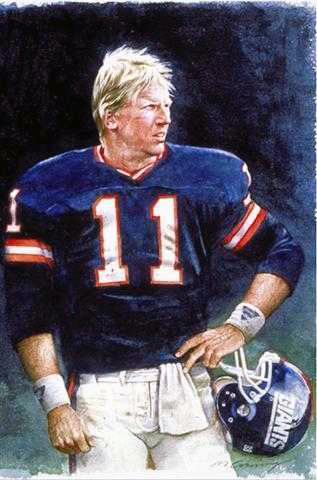This artwork is a detailed, color painting of Phil Simms, the football player. He is depicted wearing his number 11 jersey, which is predominantly blue with white and orange accents; the number 11 is shown in white with a red outline. Simms is holding a large blue helmet, emblazoned with the word "Giants" in white letters, against his right leg. His left hand rests on his waist, while his right hand hangs down by his side. He wears white wristbands with a triangular insignia or logo on both wrists. Simms' short, layered blonde hair is tousled by the wind, which is blowing to the right, the same direction he's gazing. His attire includes white pants and a small white towel hanging from his waist. The image transitions from a dark blue background at the top to a lighter blue and green gradient towards the bottom, adding depth and contrast to the composition. His face has a ruddy complexion, and the overall style of the image suggests it might be a watercolor painting.